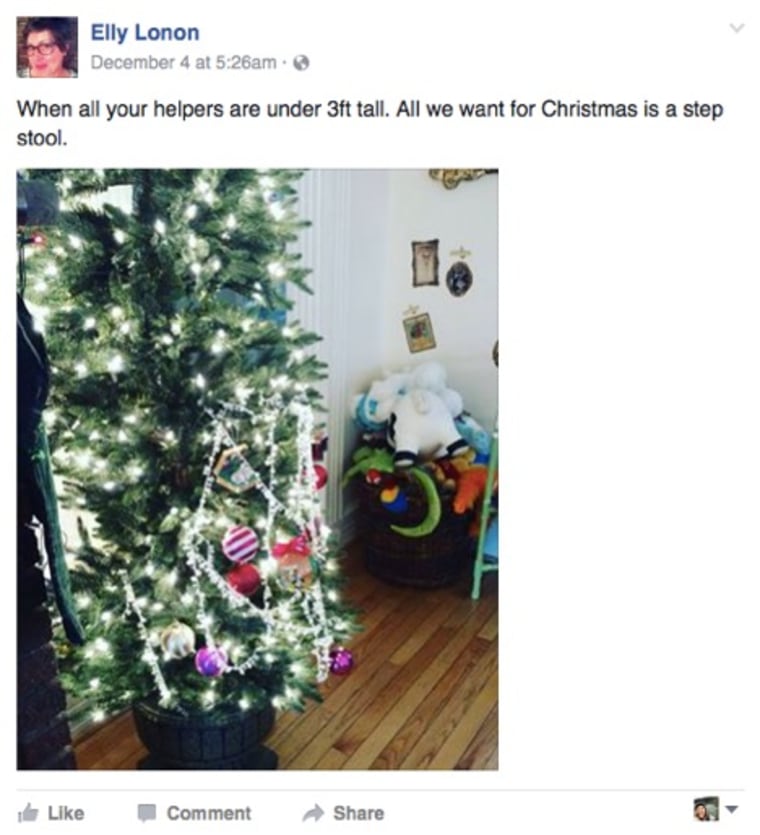In this Facebook post from December 4th at 5:26 AM, Ellie Launan—an elderly woman with black hair and glasses—shares a heartwarming scene decorated for Christmas. The post is public, indicated by a world icon next to the timestamp. Ellie's caption reads, "When all your helpers are under three feet tall, all we want for Christmas is a step stool."

The image features a festive, artificial Christmas tree adorned with twinkling lights and colorful ornaments, proudly placed atop a black stool. The setting is a cozy living room with wooden flooring. To the left of the tree, a basket brimming with toys and plushies sits in the corner. The warm ambiance is enhanced with wall decorations, including a cross and framed pictures. To the right, a stool or shelf adds to the homey atmosphere, completing the holiday scene.